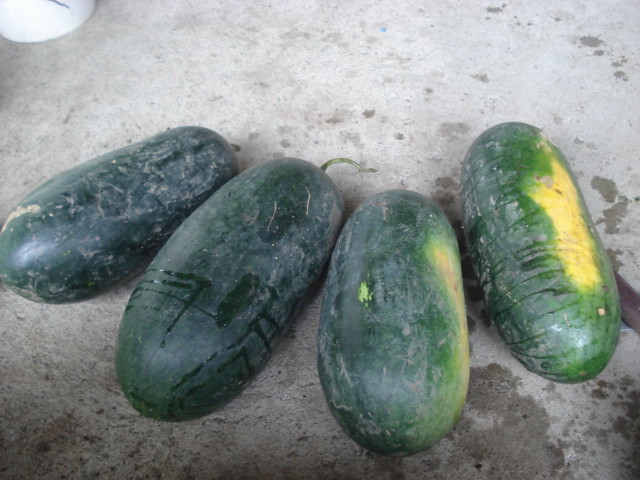The photograph captures four large, dark green, torpedo-shaped vegetables, likely cucumbers, arranged side-by-side on a concrete surface. The concrete is stained and pitted, with visible darker patches of water and drippings, particularly in the foreground. The vegetables appear slightly damp, with condensation on their skins. The one on the far left is the smallest and has a short green stem. The second vegetable is the largest and also features a visible stem. The third and fourth vegetables, positioned on the right, have lighter green and yellowish spots along their sides, with the one on the far right exhibiting a prominent yellowish flash. The arrangement of the vegetables forms a slightly curved line. A white plastic circle is visible in the top left corner of the image.